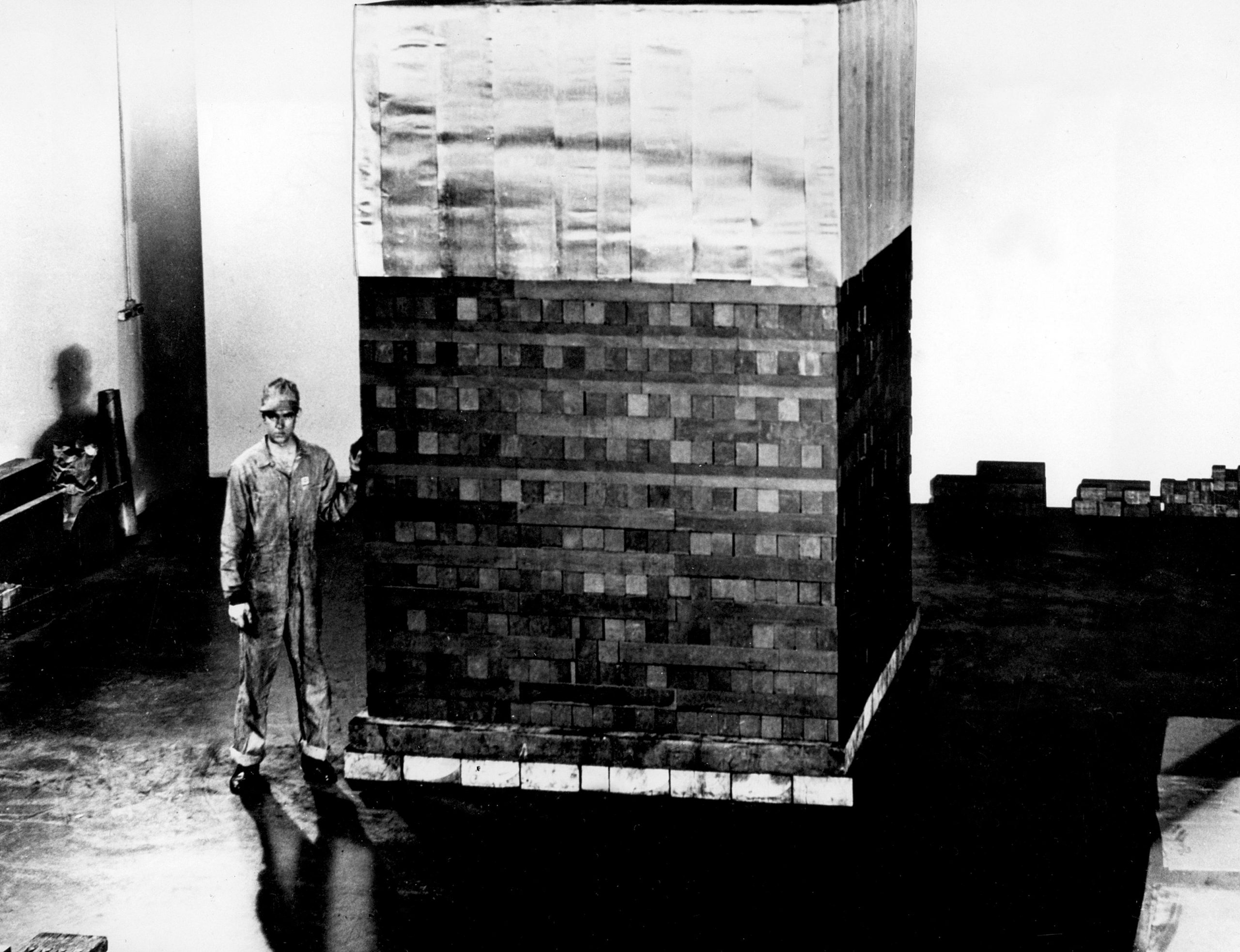This is an old-fashioned black and white photograph featuring a man standing to the left of a towering structure that resembles a giant Jenga tower made of stacked wooden blocks. The blocks are meticulously arranged in a criss-cross pattern, alternating between lengthwise and widthwise, and create a structure that is twice the man's height. The man's outfit includes a jacket, pants, and a hat, with his hands seemingly interacting with the structure. He casts a shadow on the wall to his left, adding depth to the scene. The blocks vary in shades from dark gray at the bottom to light gray at the top. To the right of the man, the floor appears dark and slightly dirty, with larger shadows extending to the right. At the bottom left of the image, a beam of light adds to the artistic composition. The background is composed of a wall that transitions from light gray to white, enhancing the contrast between the structure and its surroundings.